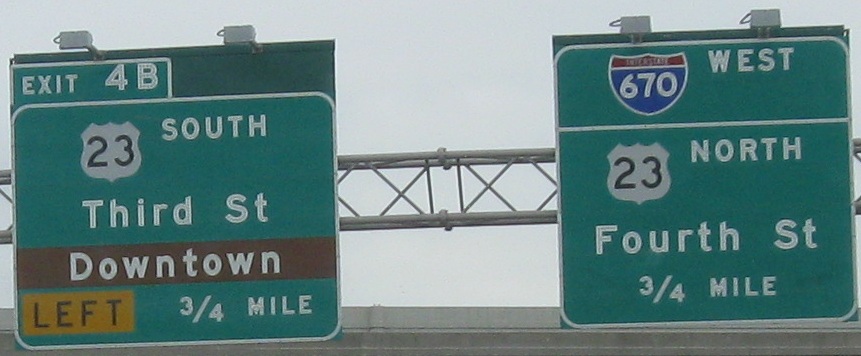This color photograph captures a pair of green roadway signs positioned above a freeway, set against a muted, gray sky, suggesting either overcast weather or poor lighting. The signs are affixed to two horizontal silver metallic beams, with an intricate arrangement of X-shaped metal bars supporting them, adding visual complexity to the structure.

The sign on the left, predominantly green with white text, reads: "Exit 4B, Route 23 South, 3rd Street." The word "Downtown" appears in a brown strip, and "Left" is displayed in black within a yellow rectangle. It also indicates the exit is 3/4 mile ahead. The sign's detail suggests it's guiding drivers towards downtown areas and emphasizing a left turn for the exit.

Adjacent to it, the sign on the right features the Interstate 670 West designation, marked within a distinct blue and red interstate shield. Below it, the sign directs towards "Route 23 North, 4th Street," also indicating a distance of 3/4 mile. Both signs are characterized by their green backgrounds and predominantly white font, serving as clear navigational aids on the freeway. The metallic beams and supporting structure, along with two small chimney-like protrusions atop the signs, contribute to the functional yet complex aesthetic of this roadside scene.